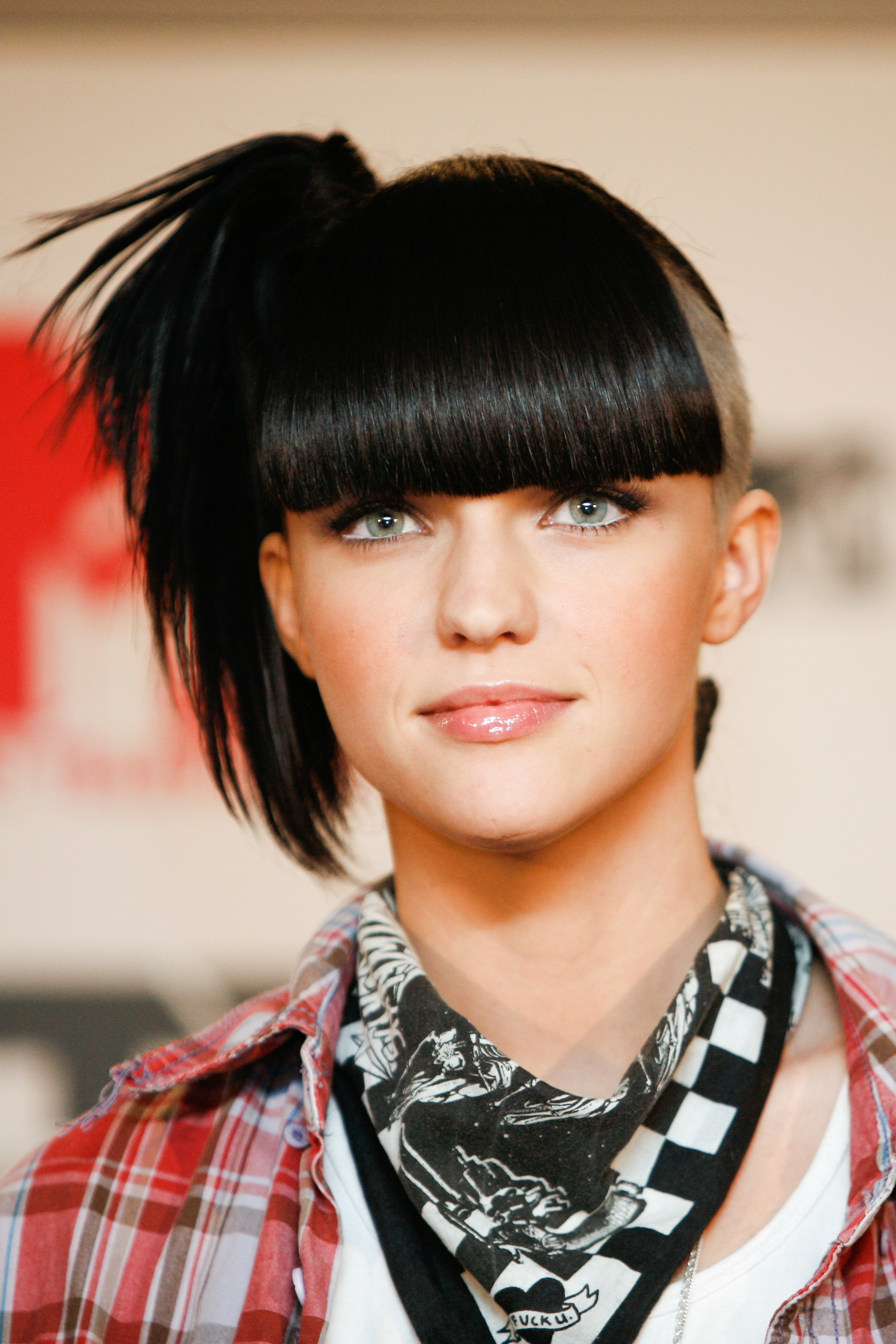This vertically aligned rectangular photograph features a young actress whose name remains unknown. The background, somewhat blurred yet distinguishable, displays a wall adorned with a mix of red and white designs along with hints of brown or black prints. The framing captures her from the chest upwards, highlighting her unique hairstyle—long black bangs cascading over her forehead, while the left side of her head is shaved, revealing tiny white or black stubs. Her hair is swept into a ponytail positioned towards the back-right side of her head.

The actress exudes a serene expression, her closed-mouth smile accentuated by shiny pink lip gloss. Her striking green eyes are directed towards the camera, creating a compelling gaze. Adorning her neck is a black and white check-patterned scarf with additional designs, notably featuring the phrase "fuck you" at the bottom. She is dressed in a plaid button-down shirt, left open to reveal a white t-shirt underneath and a prominent silver chain necklace. The visible portion of the plaid shirt exhibits a blend of red, white, and brown colors, complementing the overall casual yet edgy ensemble.